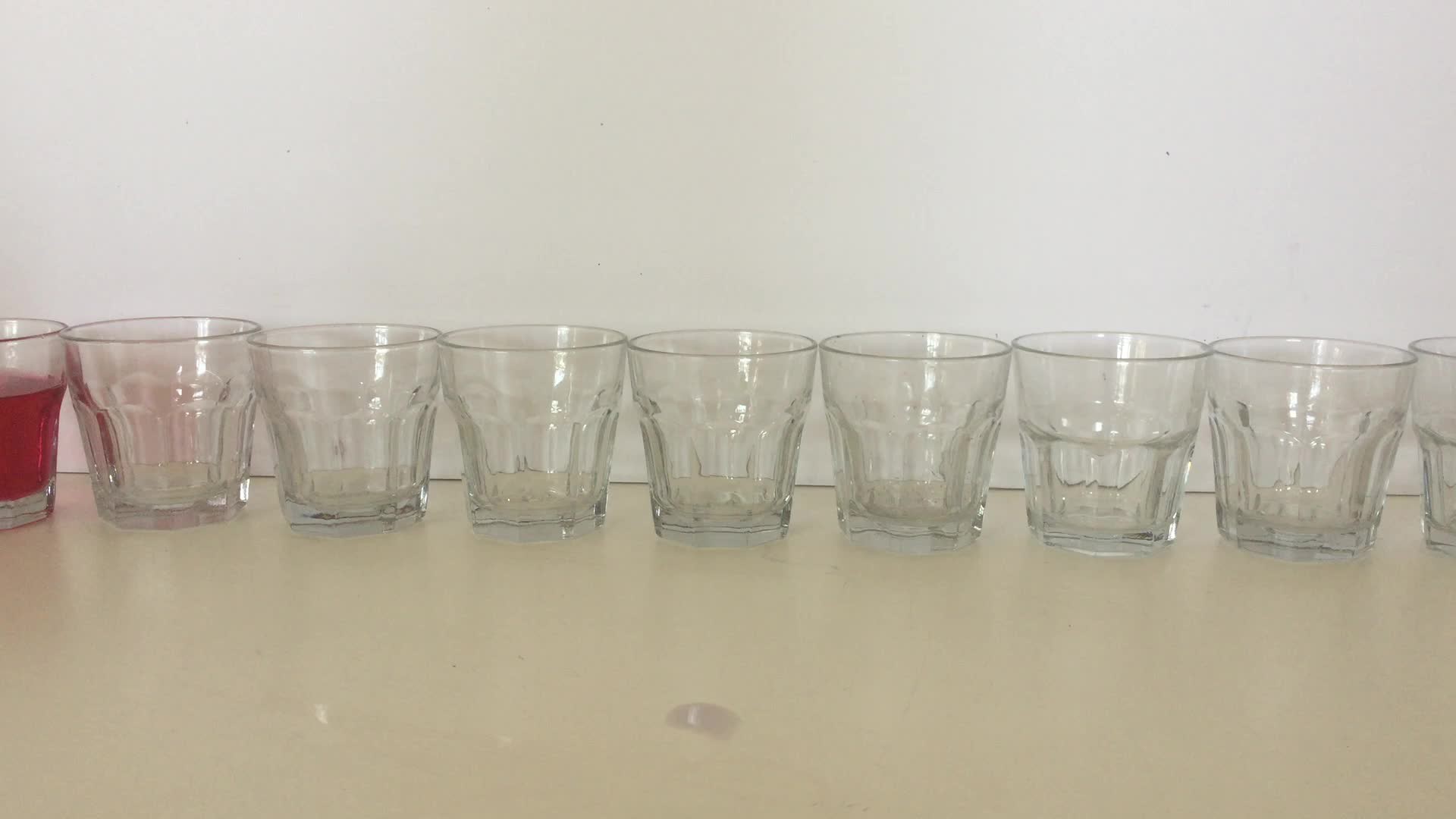This photograph features a collection of nine highball glasses arranged on an off-white, beige-colored tabletop. Against a bright white wall background, seven of these glasses are completely visible, lined up side by side and touching. All of these glasses are empty. To the left, partially cut off by the edge of the photo, is another highball glass filled to about two-thirds with a burgundy liquid. On the right side, the edge of an additional empty glass is just visible. Each glass is made of clear glass and appears clean and identical in design. In the center of the image, directly in front of the fourth glass, there is a small, irregularly shaped puddle that looks like it could be a water spill.